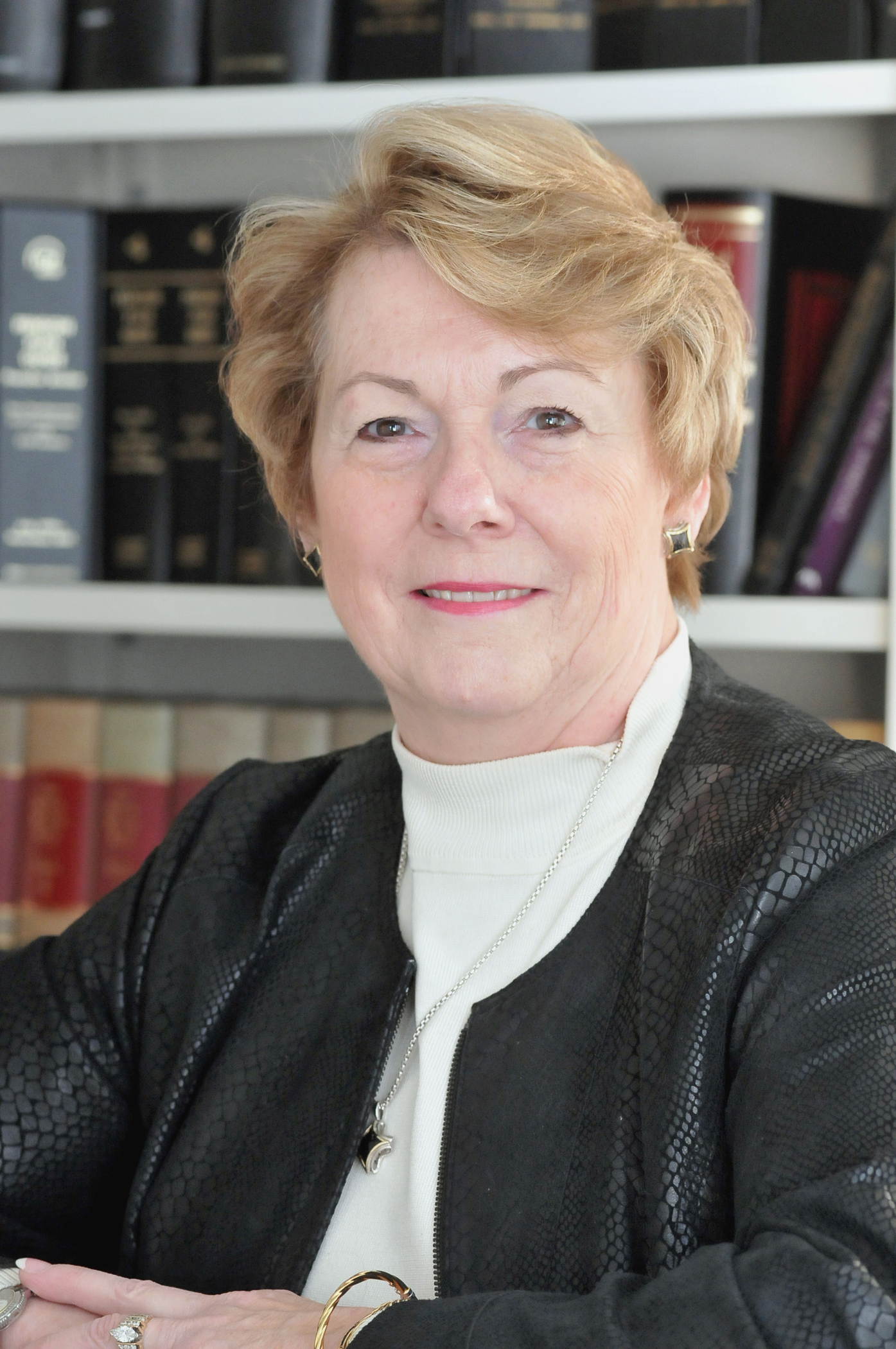The image depicts an older Caucasian woman, likely in her 60s, with short blonde hair and blue-gray eyes, seated in front of a bookshelf filled with various books in hues of black, red, and beige. She is dressed in a black snakeskin-patterned jacket over a white turtleneck shirt. Around her neck is a silver necklace featuring a star-shaped pendant. Her look is accessorized with diamond-shaped black earrings outlined in gold, a gold bracelet, and a ring adorned with a diamond. She wears pinkish lipstick and gazes straight ahead with a subtle, half-smile. Additionally, there is a hint of a silver watch on her other hand, partially visible at the bottom left corner of the image. The overall setting, coupled with her attire, suggests a professional environment.